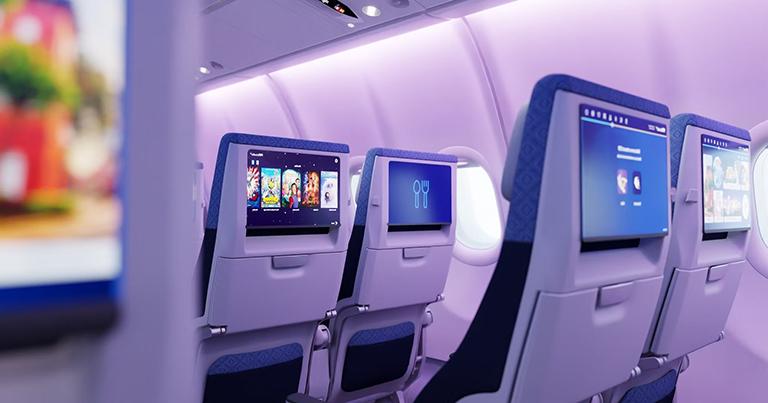The photograph captures the interior of an airplane from the point of view of a passenger seated on the left side, looking towards the right. The left side of the image blurs into a vague poster or sign with reds and greens, focusing our attention on the seats ahead. These seats show two rows of the aircraft's seating area, each featuring oval windows with open shades bathed in a soft glow. The seats are predominantly blue with some light gray plastic visible at the back. The tray tables are locked upright, and the backs of the seats have built-in screens and cloth pockets at the bottom—dark blue with a light blue stripe.

Each screen displays a different image: the closest screen presents a menu for user options or selections, the next shows a list of TV shows or movies, and the third screen, located further along, displays a clip art of a fork and spoon. The overall ambiance inside the cabin is a mix of cream and blue hues, with a notable emphasis on shades of purple and blue across the seats and the light entering through the windows. The arrangement and detailing offer a snapshot of an empty, orderly airplane cabin ready for passengers.